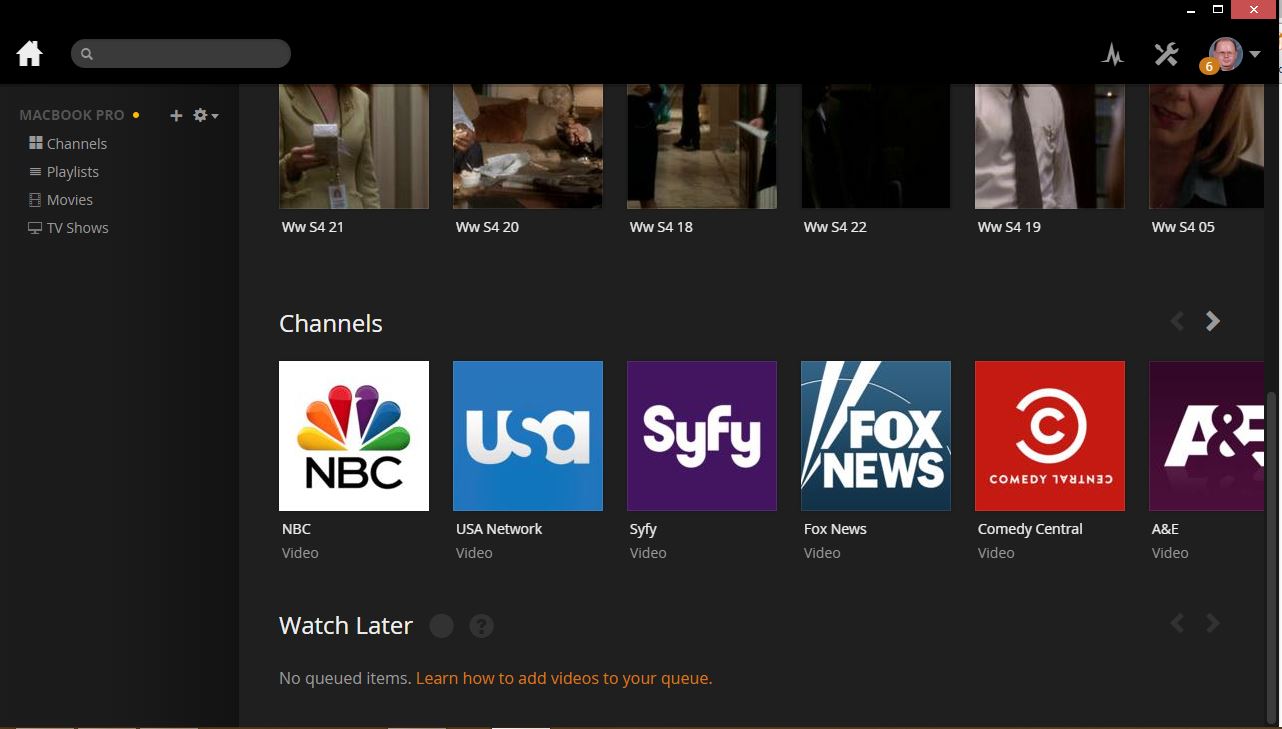The image features a gray background with a central white icon of a house, representing home, and a search bar adorned with a white magnifying glass indicating a search function. The display includes a MacBook Pro, identifiable by a highlighted yellow circle. A profile picture of a man is also present, framed by a yellow circle containing a white number six, hinting at a notification or indicator of six items. 

There are two sections detailed within the image. 

The first section lists six items, all beginning with "WWS":
1. WWS421
2. WWS420
3. WWS418
4. WWS422
5. WWS419
6. WWS405

The second section highlights six channels, each with associated video content:
1. NBC Video
2. USA Network Video
3. Syfy Video
4. Fox News Video
5. Comedy Central Video
6. A&E Video

Additionally, a "Watch Later" feature is depicted with a gray circle icon, beside another gray circle containing a question mark which likely signifies help or additional information. A notice explains "no queue items" with instructions in white and yellow for "Learn how to add videos to your queue."